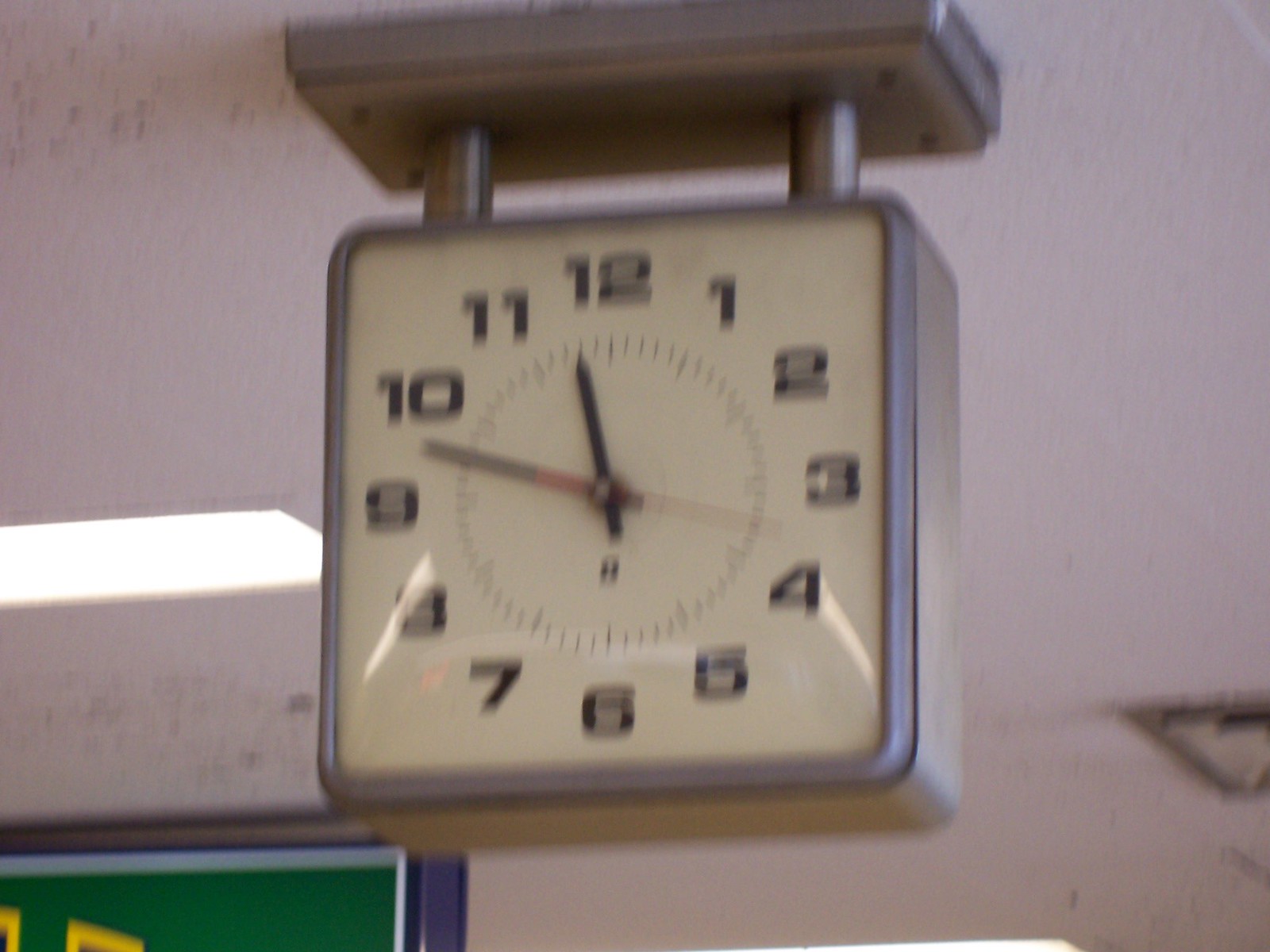This photograph features a clock hanging from a white ceiling with a speckled black pattern. The image is slightly out of focus, drawing soft attention to the centrally positioned clock. To the left of the clock, a white rectangular fluorescent light fixture is visible. In the bottom left corner, a hint of green and some silver lines suggest the presence of a poster frame or perhaps another image, adding a subtle touch of color and texture to the scene.

The main subject of the photograph is the centrally positioned clock, which dominates most of the frame. The clock itself is supported by a large silver rectangular structure, connected to two smaller silver columns that extend downward. These columns hold the square-faced clock, which prominently features a white face with black numerals. The time displayed on the clock reads approximately 11:48. The clock's hands are distinct: the hour and minute hands are black, while the second hand stands out in red.